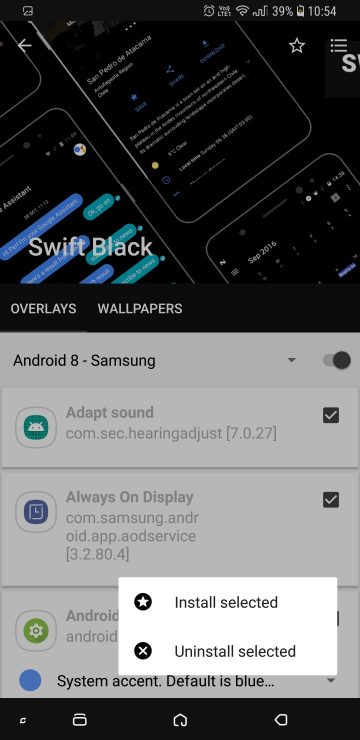The image appears to depict a photograph taken of a screen displaying multiple smaller screens, likely from cell phones, shown in a diagonal arrangement in the background. Each screen displays different random content. The image is titled "Swift Black," followed by the text "Overlays and Wallpapers." Below this title, several labels can be discerned, including "Android 8 Samsung," "Adapt Sound," "Always on Display," and partly obscured text beginning with "Android." Further down, the text reads "System Accent, default is blue." Dominating the center of the image is a large white notification bar, featuring a star icon on the left with the option to "Install Selected" and an 'X' icon on the right labeled "Uninstall Selected."